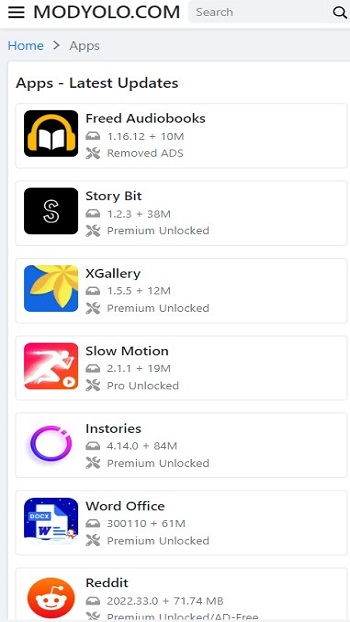This image is a cropped screenshot of the mobile app Modyolo.com, displayed on a white background. In the top-left corner, there is a black menu icon. Adjacent to this icon, the website name "modyolo.com" is prominently displayed. To the far right of this, there is a large search box featuring the placeholder text "search" in small grey letters with an accompanying magnifying glass icon symbolizing the search function.

Directly below the top bar, the navigation path is indicated, starting with "home" highlighted in blue, followed by an arrow pointing right towards the word "apps." Below this, a bold black font reads "apps, latest updates." 

The main content of the screen shows a vertical list of app icons. Each app icon is positioned to the left, with its corresponding title to the top right of the icon. Detailed information below each title includes the app size and additional features:

1. **Freed Audiobooks** - The listed details indicate the app size and note the removal of ads.
2. **StoryBit** - Below the title, it shows the app size and mentions "premium unlocked."
3. **XGallery** - Similar to the previous app, the details include the app size and "premium unlocked."
4. **Slowmotion**
5. **InStories**
6. **WordOffice**
7. **Reddit**

Each app is presented in a structured format, providing specific attributes and enhancements available on Modyolo.com.